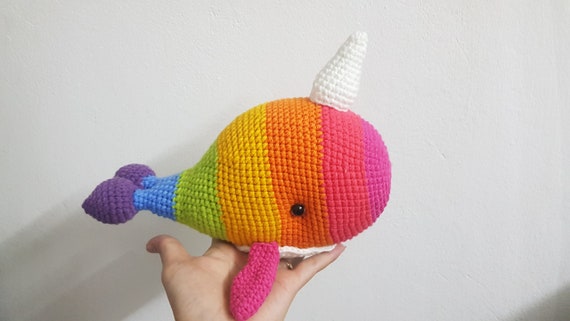The image showcases a handcrafted, rainbow-colored stuffed animal resembling a whale with a single horn, seemingly knitted from wool. Held in the left hand of a person of Caucasian descent, the whale's design includes purple tail fins, blue socks, lime green pants, and a body with vibrant stripes: pink, orange, yellow, green, blue, and purple. The whale features a distinctive white pointed horn atop its head, a black button eye on the orange strip, and small side fins extending over the person’s palm. The underbelly appears white, matching the horn. Photographed indoors against a white wall, the colorful toy, stuffed with flexible materials, casts a shadow toward the lower left, emphasizing its three-dimensionality and intricate craftsmanship.